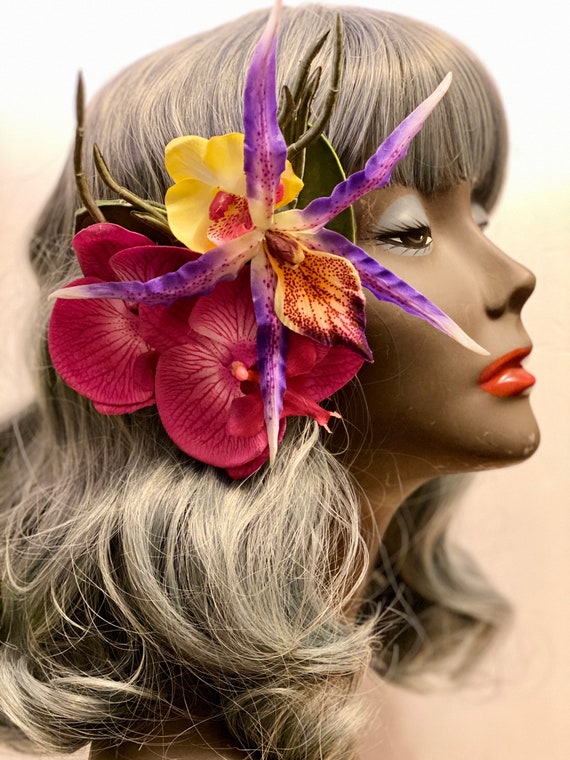The image depicts a vertically aligned rectangular picture showcasing the side profile of a female mannequin's head, turned to the right. The mannequin features tanned skin complemented by noticeable makeup, including very red lipstick and light gray eye shadow. The mannequin is adorned with a light brown to dirty blonde wig featuring straight bangs across the forehead and long, curly or wavy hair that extends past her shoulders. 

Attached to the side of her head, just above her right ear, is a complex floral arrangement. This arrangement includes two large, dark pink or red round-petaled flowers and one yellow flower. Additionally, there is a distinctive flower with a yellow pointed petal speckled with purple dots. Surrounding the arrangement are long, spiky petals that fan out in all directions, transitioning from yellow at the base to purple and then beige at the tips, with red or purple speckles adorning them. The background presents a gradient from white at the top to light brown along the sides and bottom, providing a neutral backdrop for the detailed display.